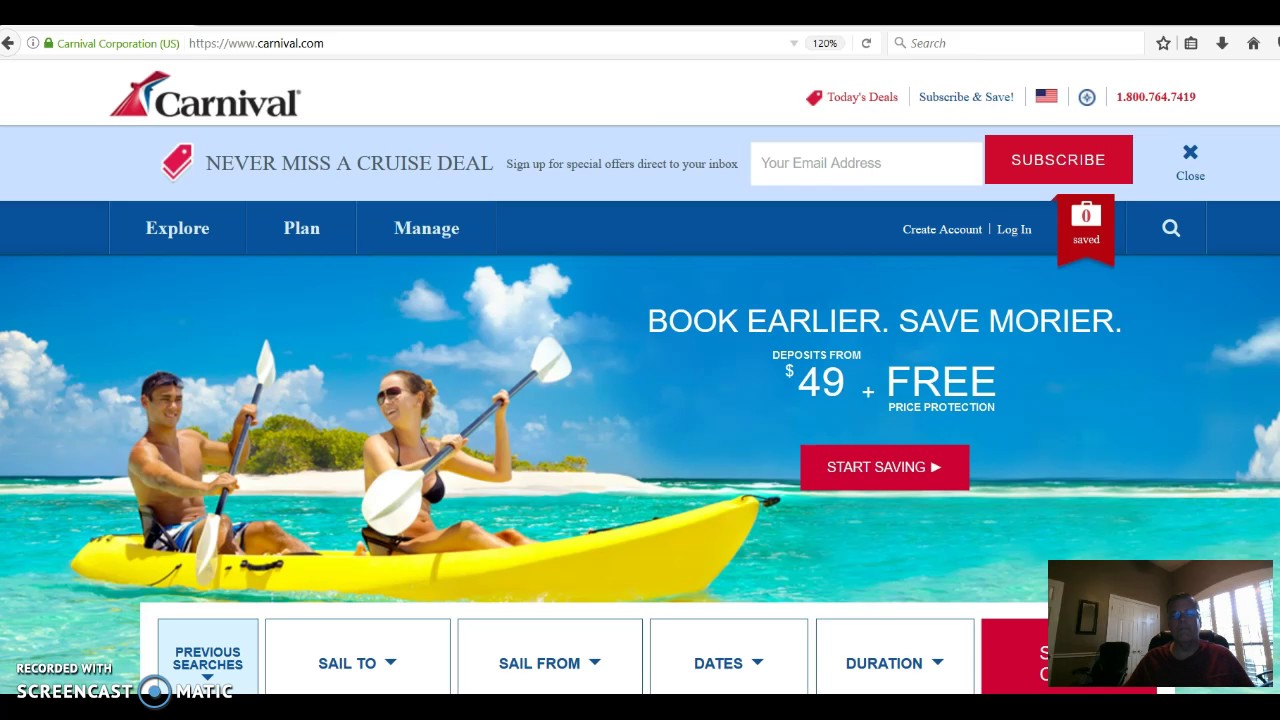Homepage of Carnival Cruise Line's website: At the top, there are several navigation links including "Today's Deal," "Subscribe and Save," and options to select a language or region. A contact number is also prominently displayed. Just below, a section encourages visitors to "Never Miss a Deal," inviting them to sign up for special offers by entering their email, with a standout red subscribe button and an option to close this element.

The main visual is a vibrant stock photo of a young man and woman paddling a canoe in crystal-clear tropical waters near the coast, embodying the adventurous spirit of the brand. Navigation links below the image prompt visitors to "Explore," "Plan," "Manage," create an account, or log in.

The central banner highlights a promotion with the tagline, "Book Earlier, Save More." It details deposits starting at $49 with free price protection. Further down, visitors are prompted to begin their searches, with a helpful screencast of a live Zoom call featuring an agent located at the bottom right of the page.